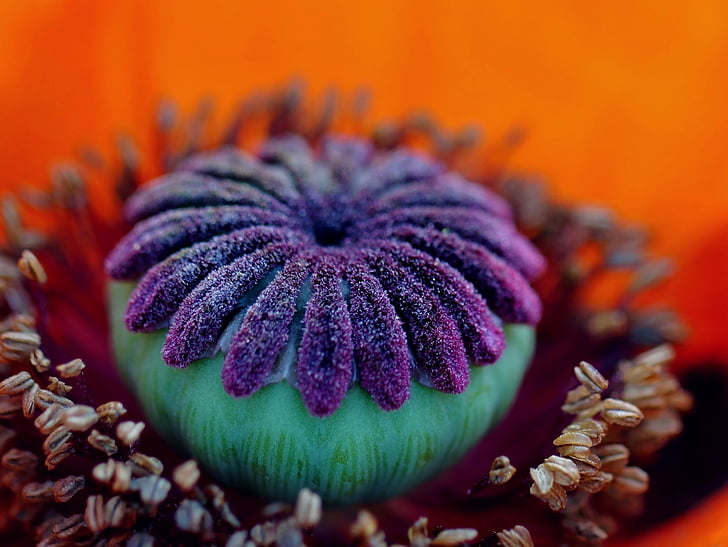The image showcases a highly detailed and vivid close-up of what appears to be a flower, most likely a poppy blossom. The central focus of the image is an intricate bloom with a base of light green or turquoise green that transitions into a vibrant purple towards the top. The purple elements are arranged like numerous tiny flower petals or fuzzy protrusions. Encircling the main structure are smaller white buds adding an additional layer of complexity. The backdrop of the photograph is completely orange, contributing to a striking contrast against the flower. The colors at the bottom of the background incorporate some hues of red and orange, enhancing the overall vividness of the image. While the setting is brightly lit with natural light, providing clear visibility, the background remains blurred to ensure the attention remains on the beautifully detailed flower in the foreground.